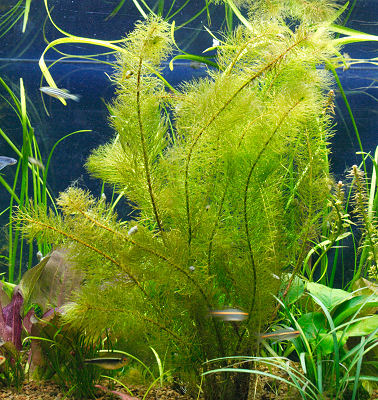The image showcases a detailed close-up of a lush, green underwater scene within a tropical aquarium. The focal point is a vibrant green plant with numerous tiny, fluffy fronds or leaves, giving it a soft, intricate texture. Surrounding this plant are various types of green vegetation, including tall, wispy grasses and long stems extending in different directions, creating a dynamic, natural arrangement. In the background, the deep blue water provides a serene backdrop for the delicate reflections of the plants and fish against the tank's glass. Scattered throughout the scene, several small tropical fish, including some that are blurry due to their fast movement, swim around. Notably, there's a little white fish in the top left corner, a darker-colored fish in the bottom left, and a few others with horizontal stripes and patches of yellow, black, or orange. Additionally, there are faint purple leaves in the bottom left corner that add a subtle pop of color. The overall image captures the lively yet tranquil essence of an underwater ecosystem rich with diverse plant life and active, minute fish.